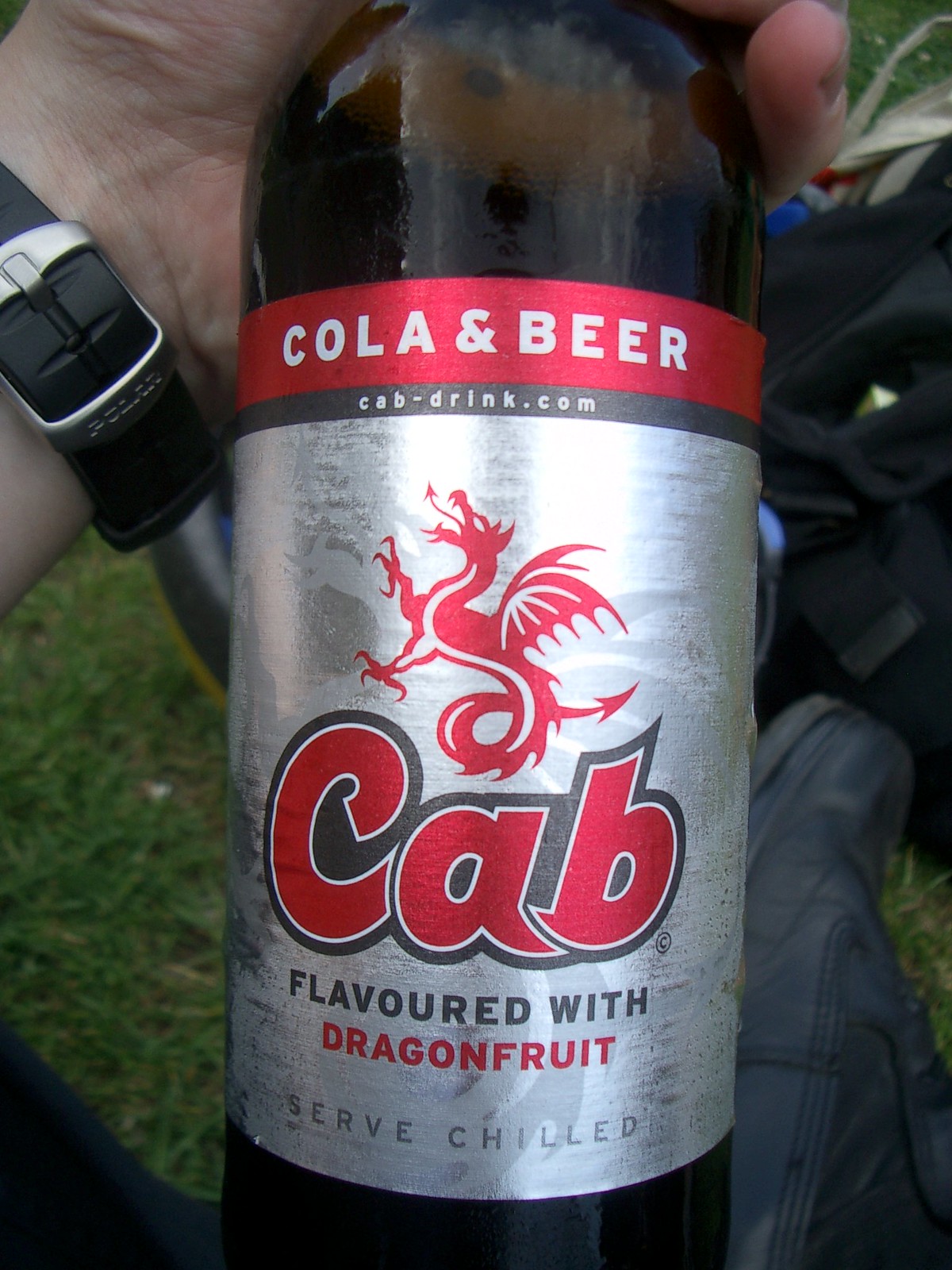In the image, there is a close-up of a hand holding a bottle from the top left, featuring a wristwatch with a black strap and silver accents. The setting is outdoors, evident by the grass visible on the bottom left and a black shoe seen on the bottom right corner. The bottle has a predominantly silver label with the text "cola and beer" written in white over a red background. Below that, it reads "cab-drink.com". The label also showcases a striking red dragon artwork, indicative of the beverage's unique flavor: dragon fruit. Additional text on the label includes "cab" in bold red text outlined in black, "flavored with dragon fruit" with "dragon fruit" in red text, and "serve chilled" in gray. The image captures natural lighting, suggesting it is taken during the daytime.